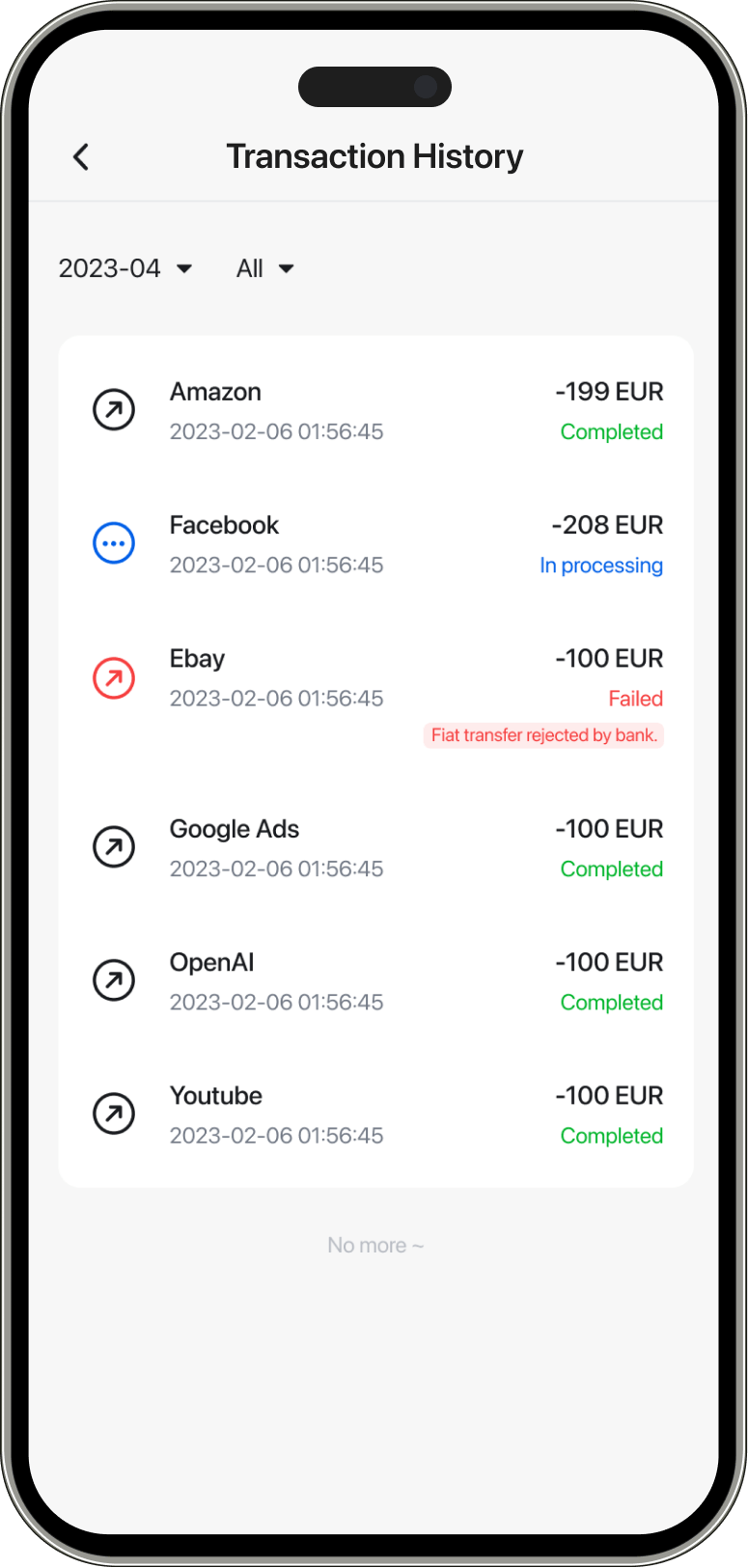This image features a black-bordered interface with a white interior background. At the top center, there is an oblong black shape containing an arrow pointing to the left. To the right of this shape, the text "Transaction History" is prominently displayed. Below this heading, towards the left side, the date "2023-04" is indicated, accompanied by a downward-pointing arrow. Nearby, the word "All" is also paired with a downward-pointing arrow.

The central portion of the image contains a list within a white box. 

1. At the top of this list, the entry reads "Amazon 2023-02-06 01:56:45 -199 EUR" with the status "Completed" highlighted in green text.
2. The next item down is labeled "Facebook 2023-02-06 01:56:45 -208 EUR", marked with "In Processing" in blue text.
3. The final entry is "eBay 2023-02-06 01:56:45 -100 EUR", with a status in red-and-white text stating "Failed: Transfer Rejected by Bank."

Each transaction entry is distinct with specific details on the date, time, amount, and current status, using color-coded indications for quick reference.